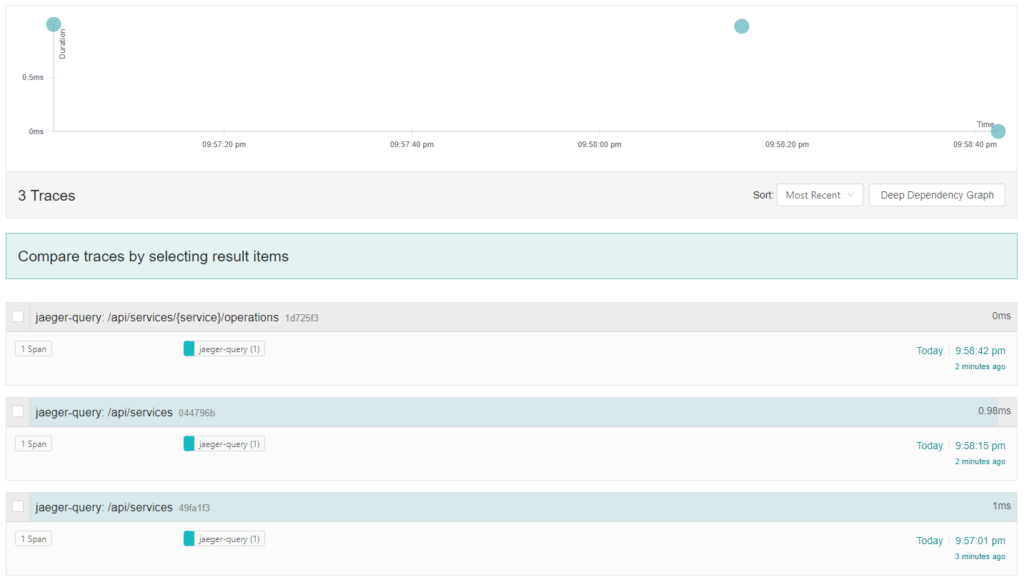**Screenshot Description: Detailed Overview**

The screenshot displays a data visualization chart where the y-axis is labeled "duration" and the x-axis represents different timestamps progressing from zero up to 9:58:40 PM. The x-axis is marked with increments of 0.5 milliseconds. Only two data points are visible on the chart, located at 9:58:20 and 9:58:40 PM.

Beneath the chart is a gray bar indicating "three traces." To the right of this bar, the options "sort," with "most recent" selected, and "deep dependency graph" are displayed. Below that, there is a blue rectangle with a prompt "compare traces by selecting result items."

Following this prompt is a gray rectangle featuring a checkbox labeled "Jaeger query," along with the identification "APA services service operations 1D725F3." To the right of this, the duration is noted as "zero milliseconds."

Underneath this, a white rectangle shows a single item: "one span," which contains a filled box labeled "Jaeger query one." To the right, it further details the timestamp "today 9:56:42 PM," indicating the record was created two minutes ago.

Next, a long blue rectangle comprises a checkbox and another "Jaeger query" entry: "API services 044796B." Below it mentions "one span," and to the right side, the recorded duration is "0.56 MS," timed at "today 9:58:15 PM," also two minutes ago.

The final portion of the screenshot highlights another blue rectangle with "Jaeger query API services 49FA113" and a corresponding duration of "one millisecond." Below this, a similar format has "one span" and "Jaeger query one," timing it at "today 9:57:01 PM," making it three minutes old.

The screenshot encapsulates a detailed, timestamped breakdown of services and their corresponding durations, useful for tracking and comparing query results over a specified timeframe.